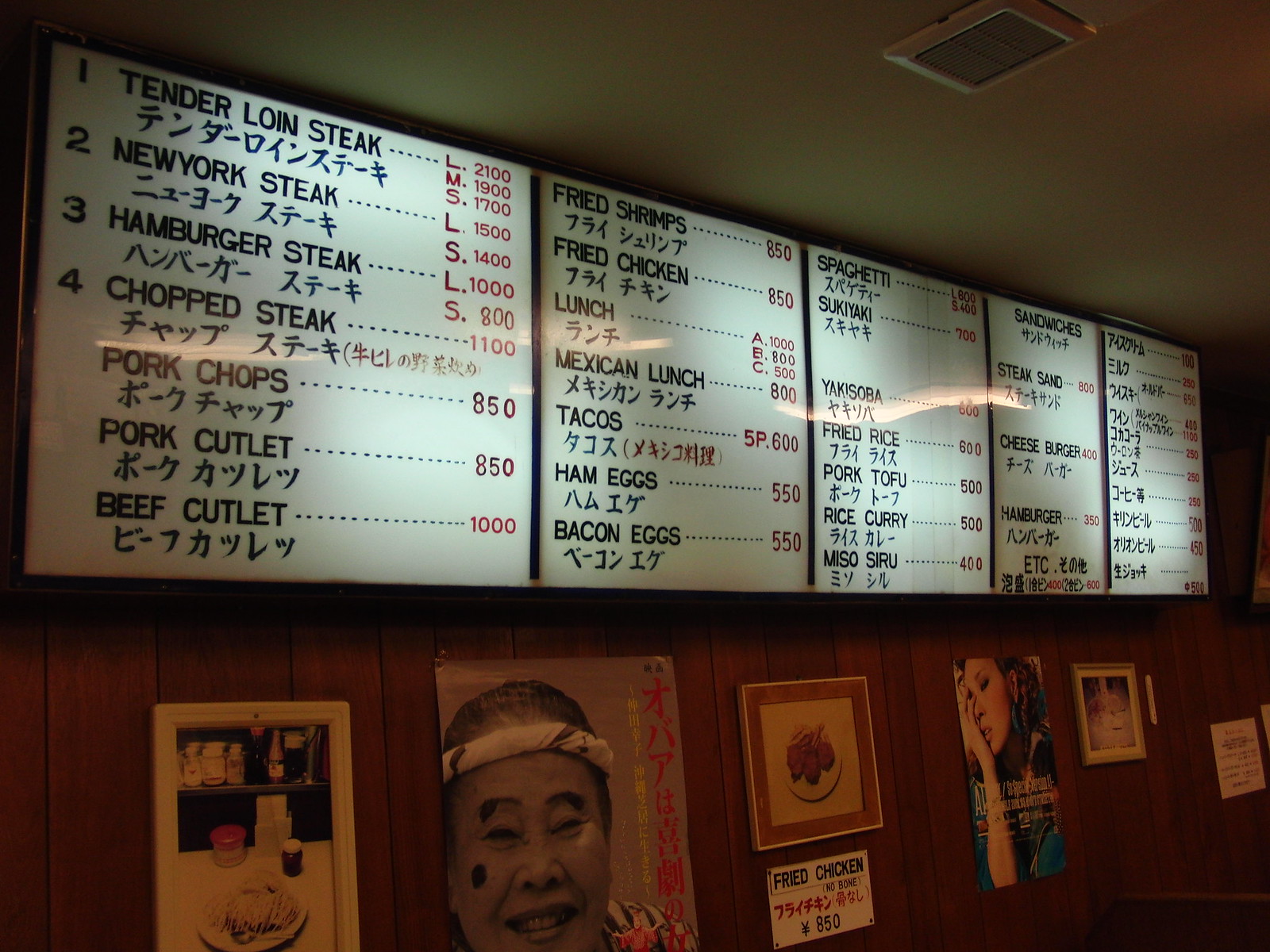The image depicts the inside of an Asian restaurant featuring an illuminated menu board comprised of five fluorescent screens displaying a diverse array of food items in both English and Asian characters. Among the menu offerings are tenderloin steak, New York steak, hamburger steak, chopped steak, pork chops, pork cutlet, beef cutlet, fried shrimp, fried chicken, various lunch combinations, and breakfast items like ham and eggs and bacon and eggs. There's also a mention of more traditional Asian dishes including sukiyaki, yakisoba, fried rice, and tofu, as well as options for spaghetti, curry, sandwiches, and salads. On one side of the menu, prices are listed next to the items, likely denoted with sizes L, M, and S. Below the menu screens, there are six pictures, including an image of a person with a headband, a framed photo associated with fried chicken, and a girl with her hand on her face. The ceiling above features some kind of lighting, casting a soft glow over the restaurant.